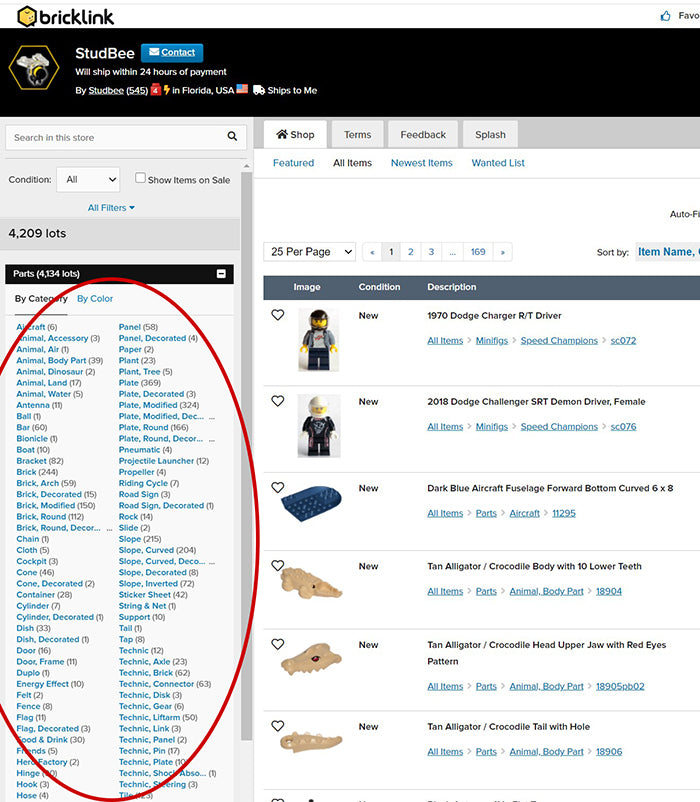This image is a screenshot from the website StudBee, indicated by the name and a yellow and black bee logo in the top left corner. The screenshot showcases various items, primarily Lego pieces, categorized and listed on the right side of the page. Among these items, two are distinctly recognizable as Lego characters, while the rest include various Lego parts, such as a tan alligator with separate components like the upper head, body, and lower teeth, each accompanied by individual images and descriptions. The page features 25 items per page, with the user currently viewing the first of 169 pages.

On the left side of the screenshot, a red circle highlights a long list of categories, which includes items like plants, trees, bells, boats, and dishes. Each category presumably contains different Lego pieces or other items, aiding users in their browsing and selection process.